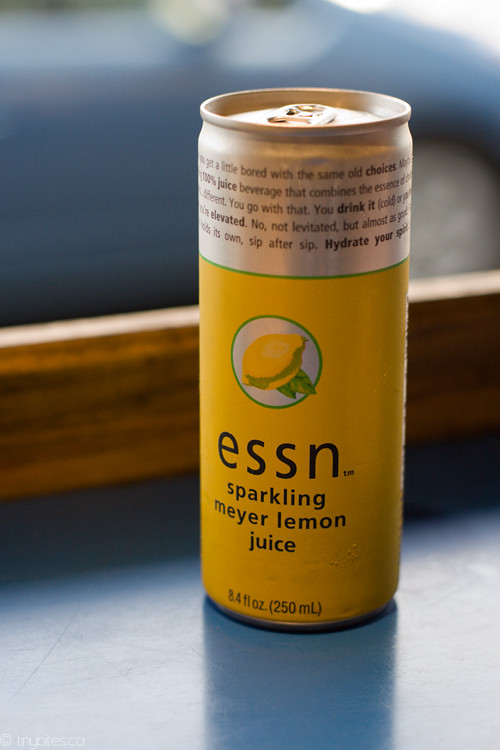Photographed here is a can of sparkling Meyer lemon juice placed on a vibrant blue tabletop. The background showcases a brown wooden trim just behind the tabletop, adding a rustic touch to the setting. Further back, a partially visible blue car with a grey section that might be the wheel subtly frames the scene. The can itself is predominantly yellow with silver accents. The label features an image of a lemon on a blue background and clearly reads: "ESSM Sparkling Meyer Lemon Juice, 8.4 fl oz." Additional text on the can invites you to break away from monotonous drink choices with this 100% juice beverage, highlighting its unique essence enjoyed best when cold. It claims to elevate (though not levitate) and maintain its refreshing quality, encouraging the drinker to "hydrate your spirit" sip after sip.